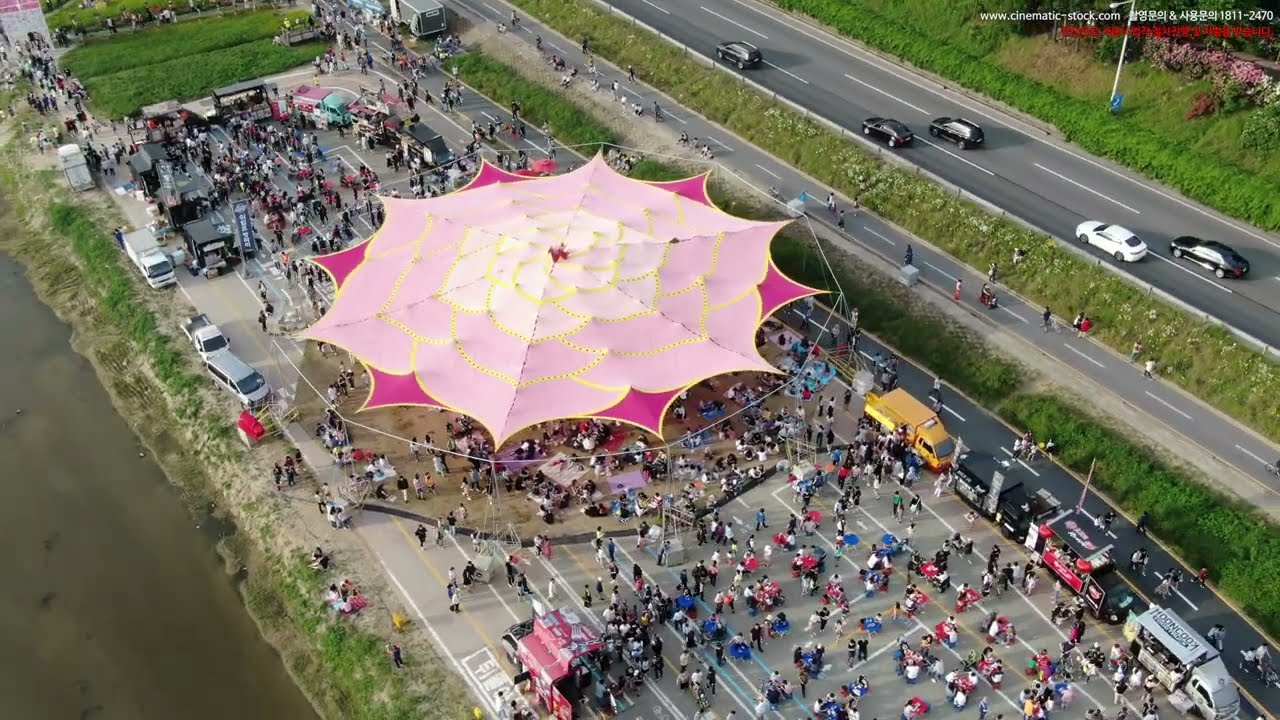The photograph captures an aerial view of a bustling outdoor festival during the daytime. In the lower left-hand corner, a brown, muddy river with a green tinge runs alongside a grassy embankment that rises to a wide paved area teeming with people. Central to the scene is a distinctive canopy shaped like a blooming flower, adorned with shades of bright pink, light pink, and golden white, supported by a white frame. Beneath and around this canopy, hundreds, if not thousands, of revelers gather, with blue and red tables scattered nearby. To the right of the canopy, numerous food trucks and other vehicles line the area. The upper right section of the image features two distinct roadways; one is possibly a walking path filled with pedestrians, while above it, a three-lane highway flows with traffic from the lower left to the upper right. The uppermost right corner includes text in white print: "www.cinematic-stock.com," followed by Korean writing and the numbers "1811-2470".